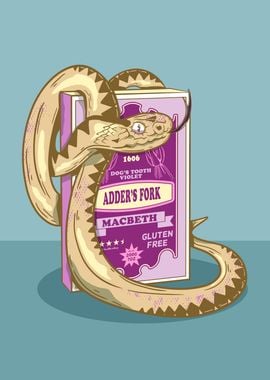The image is an artistic cartoon drawing set against a gradient teal blue background, darker at the bottom and lighter towards the top. Central to the artwork is a book colored in shades of pink, light purple, and dark purple. The book is titled "Dog's Tooth Violet, Adder's Fork, Macbeth, gluten-free," and is adorned with stars and speech bubbles. Encircling the book is a snake, portrayed in a mix of beige and dark gold colors with a pattern of diamonds on its back. The snake's tongue is sticking out, and it appears wide-eyed with flared nostrils, giving a hissing impression. Its tail extends to the right while its head is positioned prominently in the center of the image, coiled tightly around the purple book.